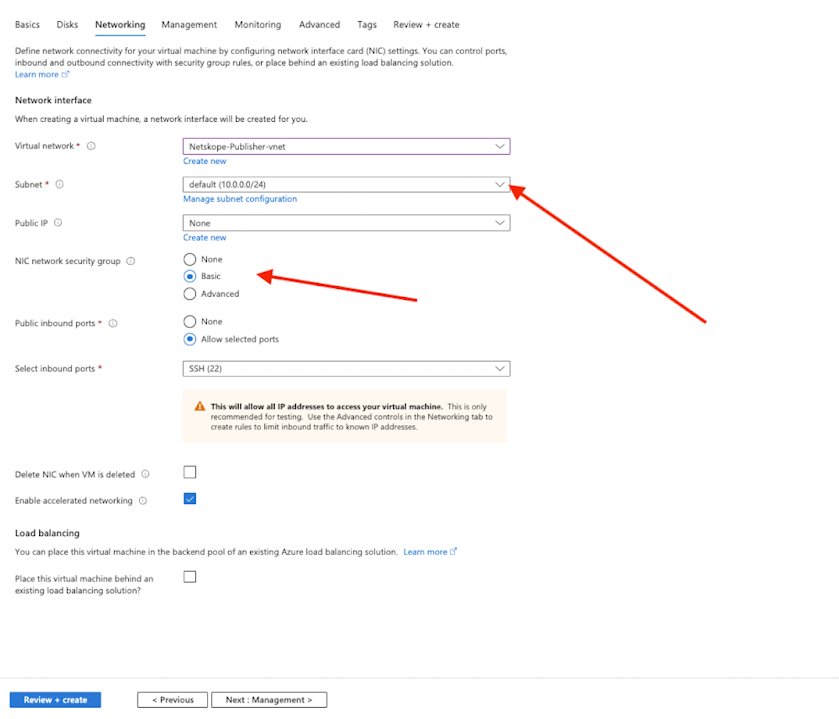**Detailed Caption:**

The screenshot captures a webpage set against a completely white background, presenting a section focused on networking settings for configuring a virtual machine. The content appears as part of a step-by-step wizard, with a navigation sidebar on the left listing various configuration topics: Basics, Disks, Networking (currently highlighted and underlined in blue), Management, Monitoring, Advanced, Tags, Review, and Create.

At the top of this section, there is a guiding text prompting the user to "Define network connectivity for your virtual machine by configuring network interface (NIC) settings." It explains that the user can manage ports, inbound and outbound connectivity using secure group rules, or position the VM behind an existing load balancing solution. A blue "Learn more" hyperlink offers additional information.

The first configuration option is labeled "Network interface." When creating a virtual machine, a network interface will be automatically generated. The "Virtual network" field shows "netscope-publisher.vnet" with a nested "Subnet" field displaying "default (10.0.0.0/24)." A blue "Manage subnet configuration" hyperlink is available below this information. Adjacent to the virtual network field is a "Create new" hyperlink, also in blue.

Next, the "Public IP" configuration is set to "None," with a blue "Create new" hyperlink next to it for adding a public IP.

The "NIC network security group" section offers three security group options: None, Basic, and Advanced. The "Basic" option is preselected, marked with a blue dot. Diagonally pointing red arrows guide the viewer's attention towards the "Subnet" dropdown and the selected "Basic" option.

The "Public inbound ports" section allows the user to choose between "None" and "Allow selected ports," with "Allow selected ports" being preselected with a blue circle. The following "Select inbound ports" dropdown box lists "SSH (22)," and an adjacent orange alert icon warns that selecting this option will permit all IP addresses to access the virtual machine, suitable only for testing purposes. It advises using advanced controls in the networking tab to restrict inbound traffic to known IP addresses.

The option "Delete NIC when VM is deleted" remains unchecked.

The "Enable accelerated networking" option is checked, indicated by a blue checkmark.

Further down, the "Load balancing" section states that the virtual machine can be placed in the backend pool of an existing Azure load balancing solution. A blue "Learn more" hyperlink offers more details. Below this, a checkbox asks, "Place this virtual machine behind an existing load balancing solution?" which is currently unchecked.

Finally, the bottom of the page provides navigational buttons: a blue "Review and create" rectangle, and grey "Previous" and "Next: Management" buttons, guiding the user to the next steps in the setup process. There is no other text visible on the page.